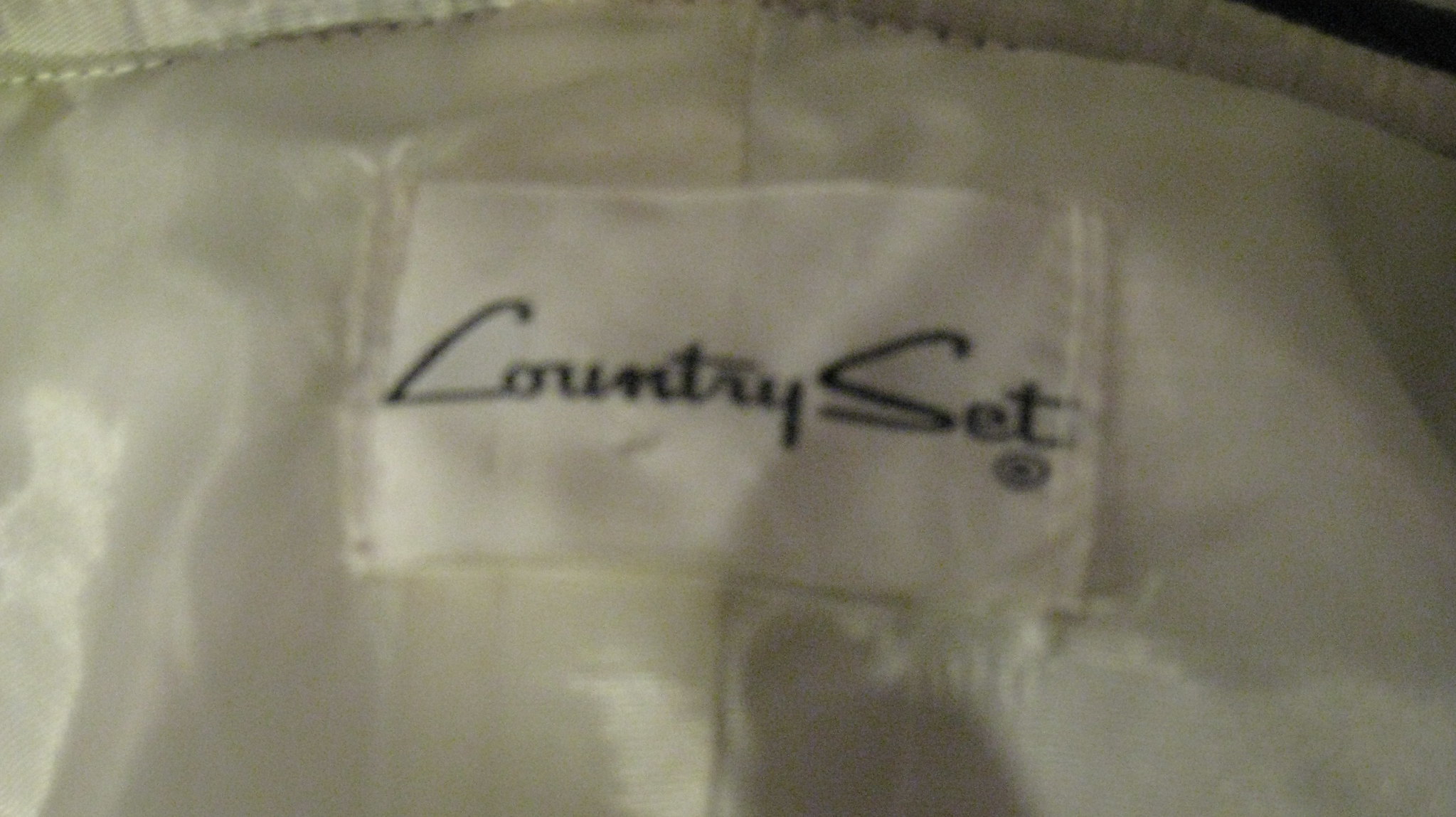This close-up photograph features a detailed view of a label sewn onto a piece of fabric. The background is predominantly white, with a noteworthy black triangle situated in the upper right-hand corner. The central focus is a white rectangular label, bordered on both the left and right sides by two rows of white stitching that attach it securely to the underlying fabric.

Midway across the label, a stylish black cursive script spells out "Country Set." Directly beneath the "T" in "Country," there is a small black circle containing a black "R," indicating a registered trademark. At the top left portion of the image, a line of white stitching extends almost to the center before a patch of plain white fabric interrupts it. The stitching then continues uninterrupted all the way to the right edge of the photo.

The fabric to which the label is attached exhibits slight ripples and appears to be made of a white satin-like material, contributing a subtle sheen to the overall visual texture of the image.